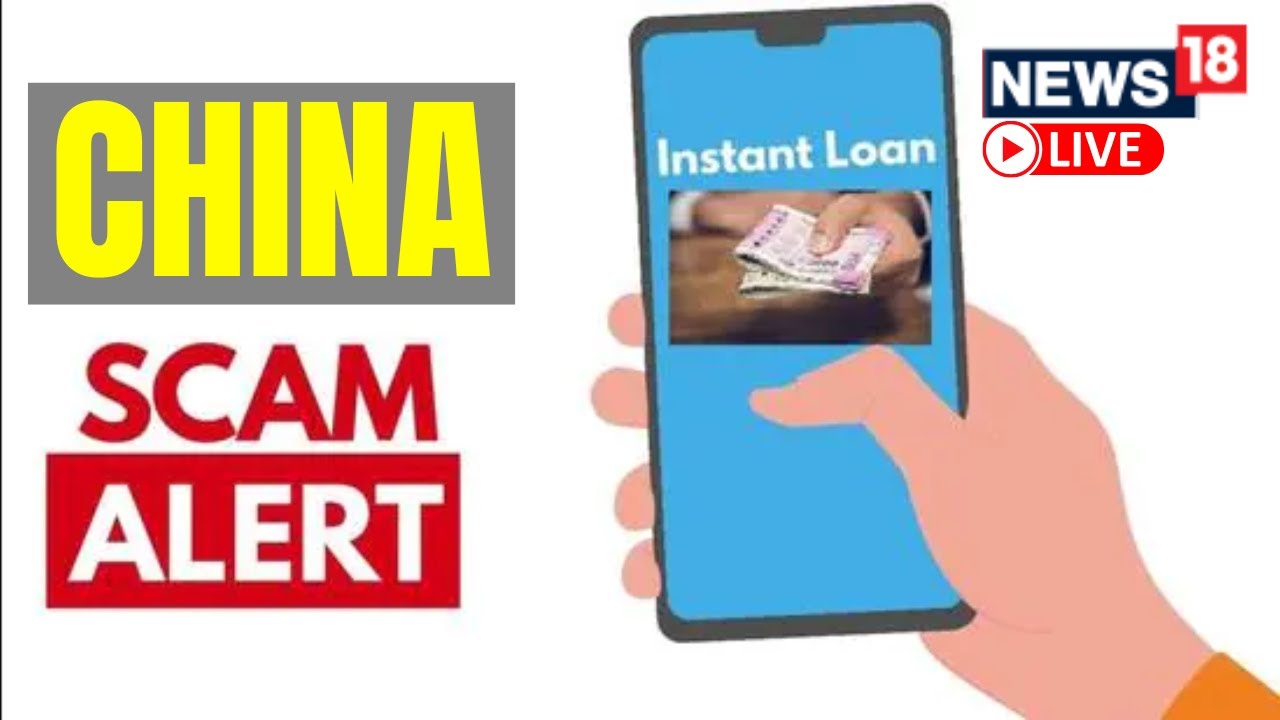This is a horizontally-oriented, computer-generated graphic typically viewed on a computer or smart device. Against a white background, a thin black line runs vertically along the left edge. The main elements include a central gray rectangle featuring large, bold yellow letters spelling "China," with the word "scam" in red text beneath it. Below "scam," a red rectangle contains the word "alert" in white letters.

At the center of the image, there is a computer-generated depiction of a hand, colored in a salmon-peach hue, with an orange sleeve extending to the wrist. The hand grasps a smartphone with a blackish-gray border and a blue screen displaying the words "instant loan" in white text alongside an image of someone holding money.

In the upper-right corner, a black rectangular box contains the word "news" in white letters. Beneath this, a smaller red rectangle displays the number "18" in white, with the word "live" in white text below it on a red background, accompanied by a small play button icon.

This graphic appears to be a warning message, possibly related to a news alert about a scam originating from China.